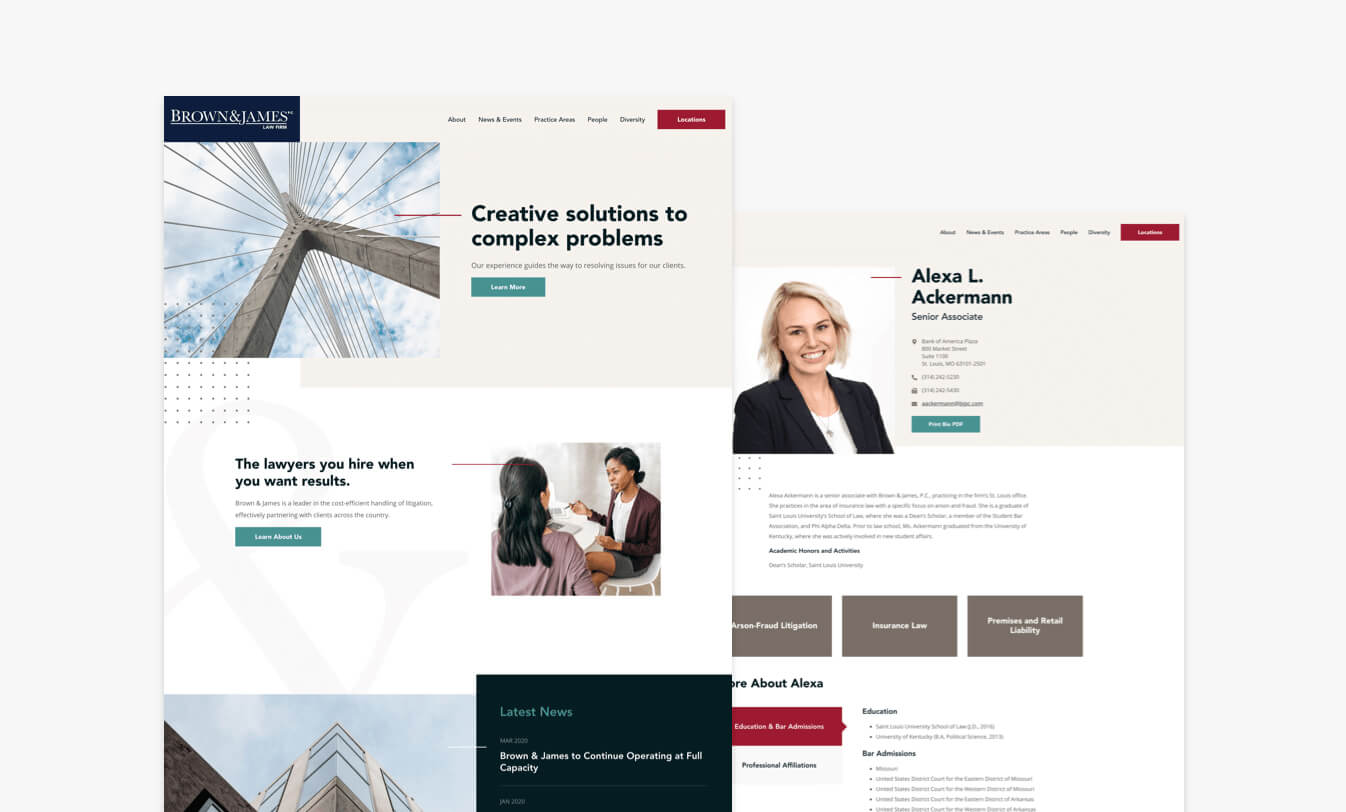The image displays two overlapping pages with a variety of elements. On the top page, positioned on the left, the top corner reads "Brown and James." Adjacent to this title is a striking photograph of a bridge, taken from an angle beneath it, showcasing one of the bridge's support structures and numerous connecting lines or ropes. The right side of this photo is overlaid with the text "Creative solutions to complex problems," highlighting the company's approach to resolving client issues. Midway down, a blue box invites engagement with "Learn More," accompanied by a subtext, "The lawyers you hire when you want results."

Additionally, this top page declares that Brown and James are leaders in cost-efficient legislation handling and effective client partnerships across the country. Another blue box towards the bottom right reiterates the call to "Learn About Us."

Further to the right, the image captures the interaction between two women. One has her back to the camera and is dressed in a sleeveless grey top with red accents. She faces another woman sitting in a white chair, who is clothed in a white shirt, grey skirt, and deep brown jacket. This second woman holds a pen and works at a table with a laptop, indicating an engaging discussion between the two.

In the lower left portion of the page, a partially visible building set against the sky is cut off mid-image. To the image’s right, text headlines "Latest News - March 20," followed by a blurry 2000 and white text reading "Brown and James to continue operating at full capacity." Below, another date, "Jan," is partially discernible.

On the second, slightly visible page, a profile reveals the image of a smiling white woman with white hair, dressed in a black suit jacket and white shirt, accessorized with a necklace. She is identified as "Alexa L. Ackerman, Senior Associate," with contact details including an address, phone number, fax number, and email, along with options to print or save a PDF.

A brief, blurry biography follows, marked by the bold heading "Academic Honors and Activities." Beneath this, three brown boxes with white lettering are labeled "Arson Fraud Legislation," "Insurance Law," and "Premises and Retail Liability." Below these boxes, text on a white background reads "More about Alexa," succeeded by a red box with "Education" and "Bar Admissions." Professional affiliations appear under this main section, detailed with bullet points, although the text remains unclear due to blurriness.